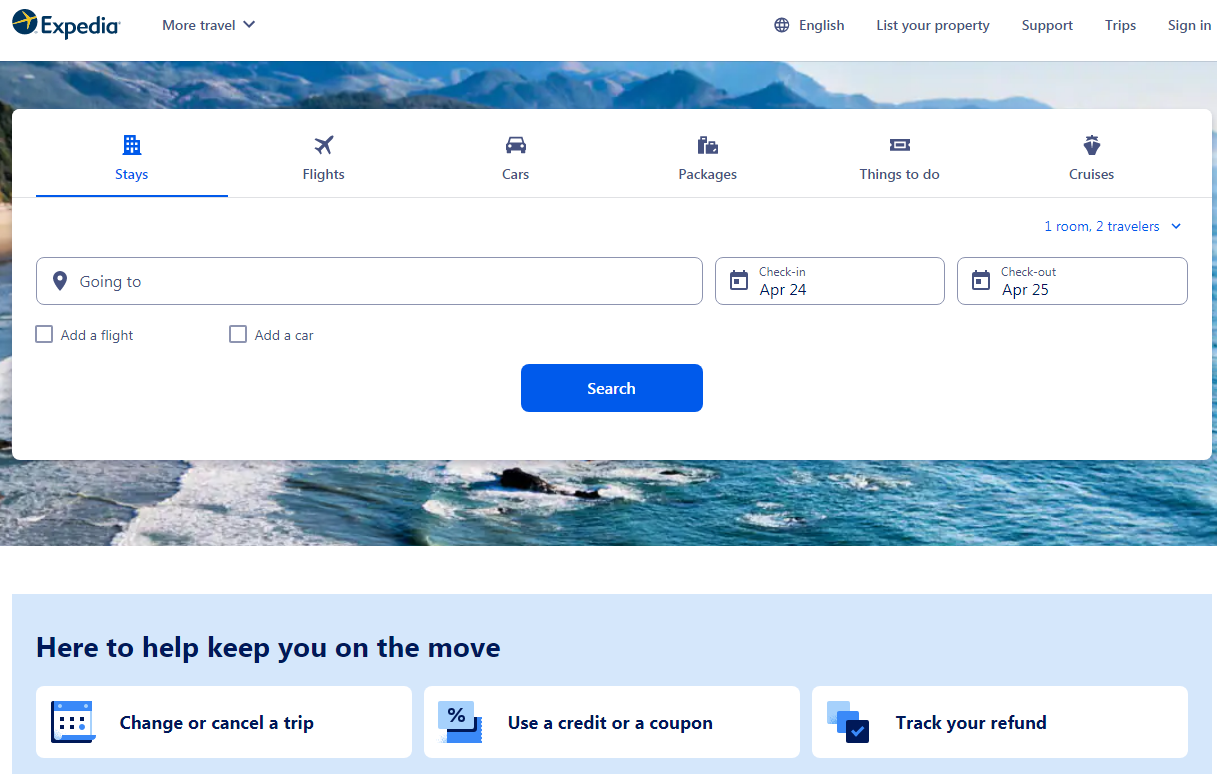This image is a screenshot of the Expedia website interface. At the top left, the Expedia logo - a circle with an airplane flying through it - prominently appears next to the Expedia name. To the right, a navigation bar displays options: "More travel," "Sign in," "Trips," "Support," "List your property," and a globe icon adjacent to the word "English." 

Centered on the page is a large white rectangular section with several navigational tabs lined horizontally across the top. From left to right, these tabs read: "Stays," "Flights," "Cars," "Packages," "Things to Do," and "Cruises," with "Stays" highlighted in blue and underscored.

Below these tabs are three entry boxes for search details. The first box is labeled "Going to." The next two smaller boxes are for check-in and check-out dates, specifically: "Check-in, April 24th," and "Check-out, April 25th." A prominent blue "Search" button is situated at the bottom of this section.

At the very bottom center of the image, a reassurance headline states, "Here to help keep you on the move." Flanking this, on the bottom left, are options to "Change or cancel a trip," in the middle, "Use a credit card or coupon," and on the bottom right, "Track your refund."